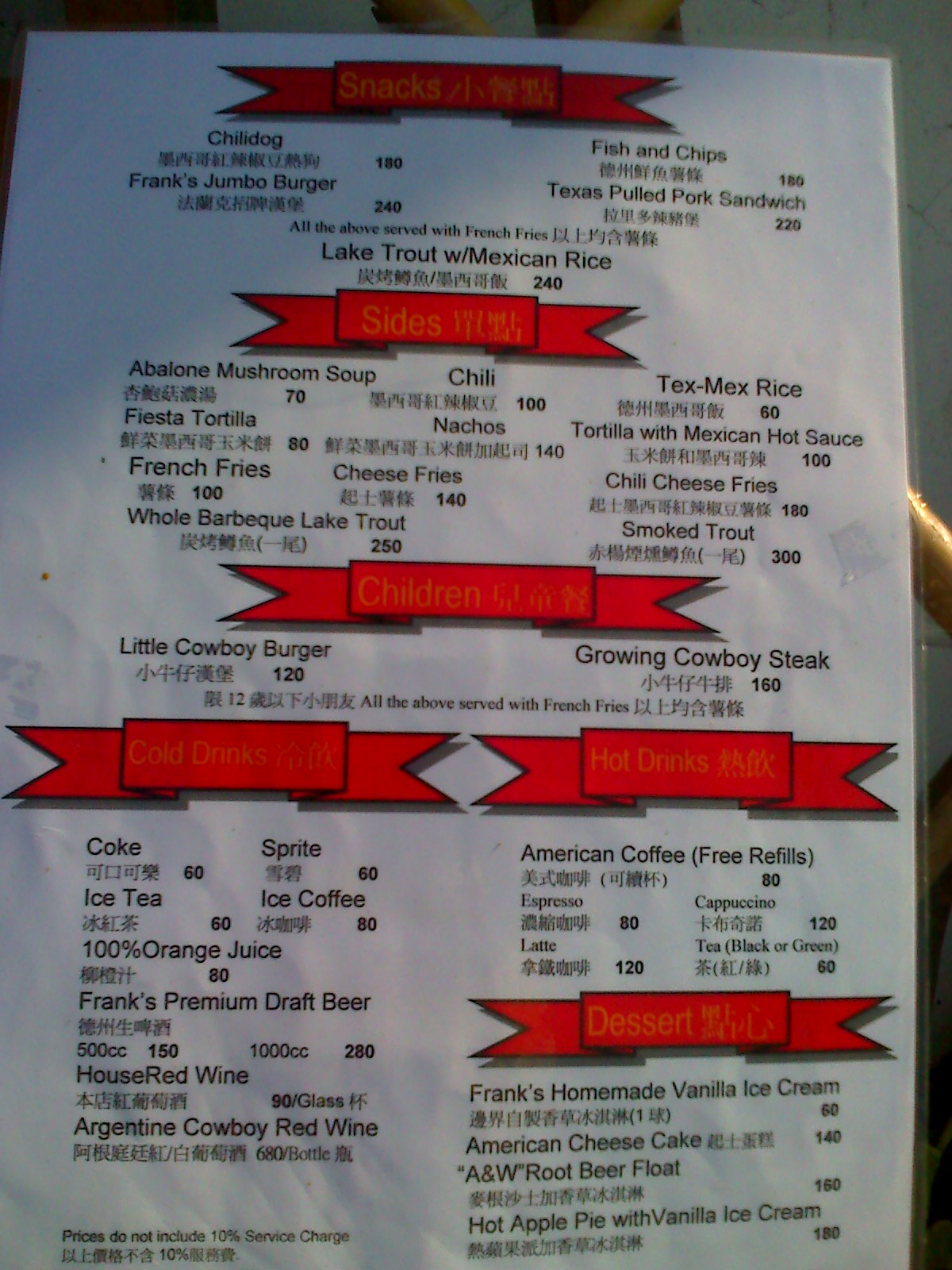The image features a menu displayed on a white piece of paper set against a slightly gray background. At the top of the picture, a hint of brown can be seen. The right side of the image includes a partial view of someone's hand and fingers holding the menu. The menu itself is adorned with red accents, including small flags, that categorize different types of dishes.

The menu lists an array of mouth-watering options, starting with savory items such as Chili Dogs, Frank's Jumbo Burger, Fish and Chips, and a Texas Pulled Pork Sandwich. Seafood lovers can indulge in Lake Trout Mexican Rice, Abalone Mushroom Soup, Smoked Trout, and Whole Barbecue Lake Trout. Classic comfort foods and Tex-Mex favorites include Fiesta Tortilla, Nachos, French Fries, Cheese Fries, Tex-Mex Rice, Tortilla with Mexican Hot Sauce, as well as Chili Cheese Fries.

For meat enthusiasts, there's a Little Cowboy Burger and a Growing Cowboy Steak. Beverage choices range from soft drinks like Coke, Sprite, Iced Tea, Iced Coffee, and 100% Orange Juice to alcoholic selections such as Frank’s Premium Draft Beer, House Red Wine, and Argentina Cowboy Red Wine. American Coffee with free refills is also available.

Dessert choices don't disappoint with Frank's Homemade Vanilla Ice Cream, American Cheesecake, A&W Root Beer Float, and Hot Apple Pie paired with Vanilla Ice Cream rounding off the delectable offerings.